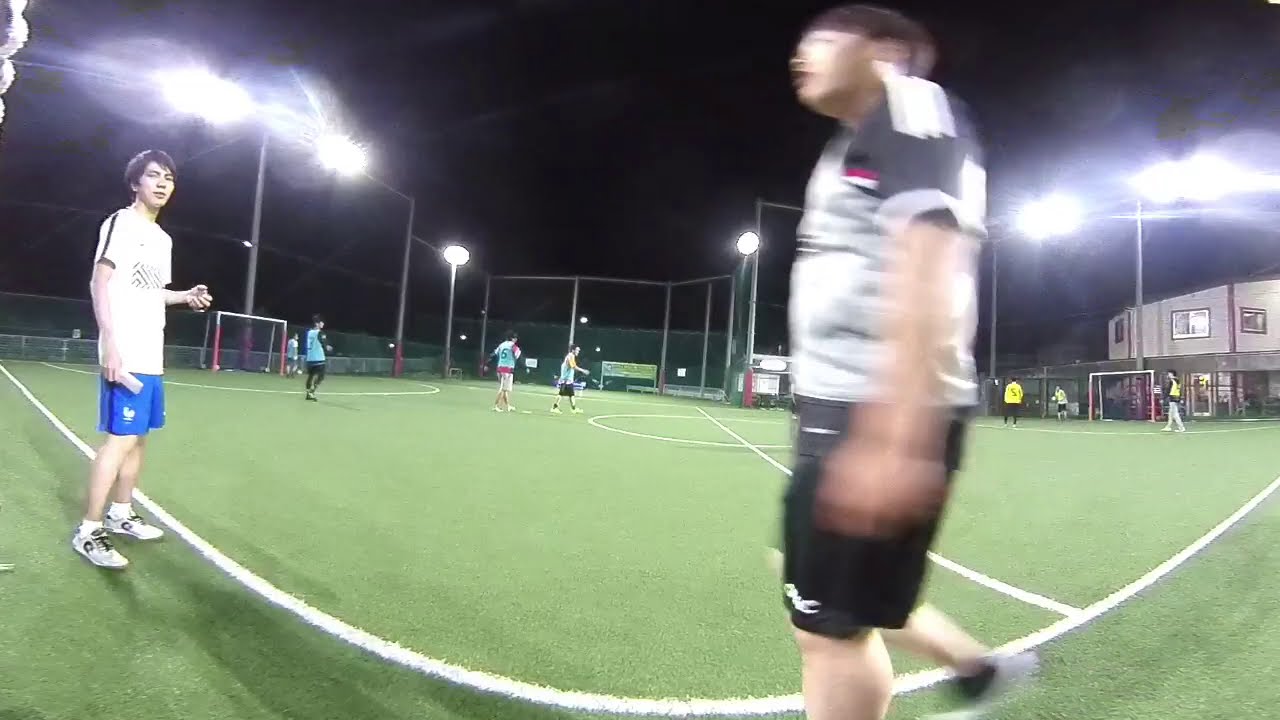In the image, we see an outdoor soccer field illuminated under the night sky, creating a striking contrast with the darkness above. The field, lush and green, is enclosed by fencing and features multiple goalposts scattered across it, indicating areas designated for practice. The vibrant setting is bustling with activity, as around 20 young athletes, seemingly in their 20s or younger, are scattered across the field, many dressed in a variety of athletic wear, with some notable details standing out. One male, clearly Asian, is sporting a yellow t-shirt, blue shorts, and white sneakers accompanied by low-cut socks. Another potential teenager is clad in black shorts paired with a gray and black t-shirt. The action and energy on the field are captured by a GoPro, creating a unique, slightly distorted perspective that makes it seem as though you're looking into a globe.

To the right side, a blurred figure—wearing a white top and black shorts—dominates the foreground, as though they just walked past the camera. Nearby, a kid in a white t-shirt and blue shorts stands, appearing to observe the action. The stadium's powerful floodlights create a halo effect with their brightness, adding to the dynamic atmosphere. Beyond the field, various structures are dimly visible; one building, possibly a facility entrance or a souvenir shop, is lit up and stands on the far right, adding depth and context to the lively scene.